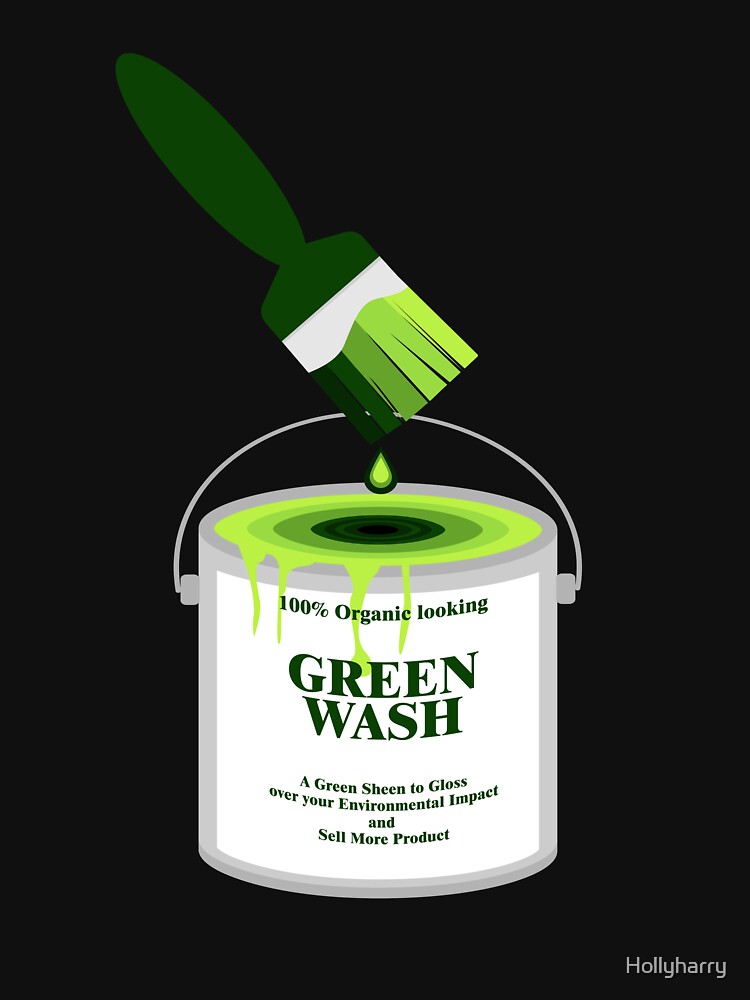The image is a vertically oriented cartoon vector art with a solid black background. At the center bottom, there is a light gray (silver) paint can with a white label. The label reads in green lettering, "100% Organic Looking Green Wash, a green sheen to gloss over your environmental impact and sell more product." The paint can is open and filled with various hues of green paint, which appear to be overflowing and dripping down the side. Positioned above the paint can at a 45-degree angle is a green-handled paintbrush. The bristles of the brush are depicted in a gradient from dark green to light green, with a drop of green paint dripping from the bristles into the open can. This image satirizes superficial environmental claims by companies. In the bottom right corner, there is a credit that reads "Holly Harry."